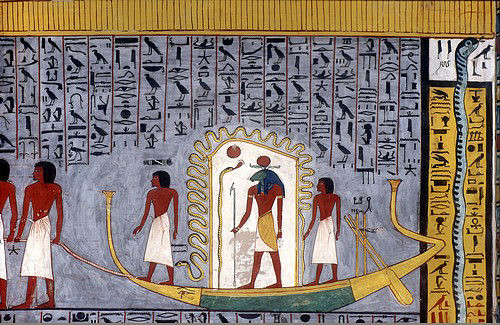This detailed depiction of Egyptian art features a substantial gray background, framed by a light brown border embellished with fine black lines, resembling wooden planks. At the center of this composition is a prominent gray expanse filled with intricate drawings. Standing out among the depictions is a large white doorway, through which a figure with the body of a man but the face of an animal is entering, holding a long staff. Inside, several other figures with human faces are visible, adorned in traditional white waist wraps, enhancing the authenticity and cultural significance of the artwork.